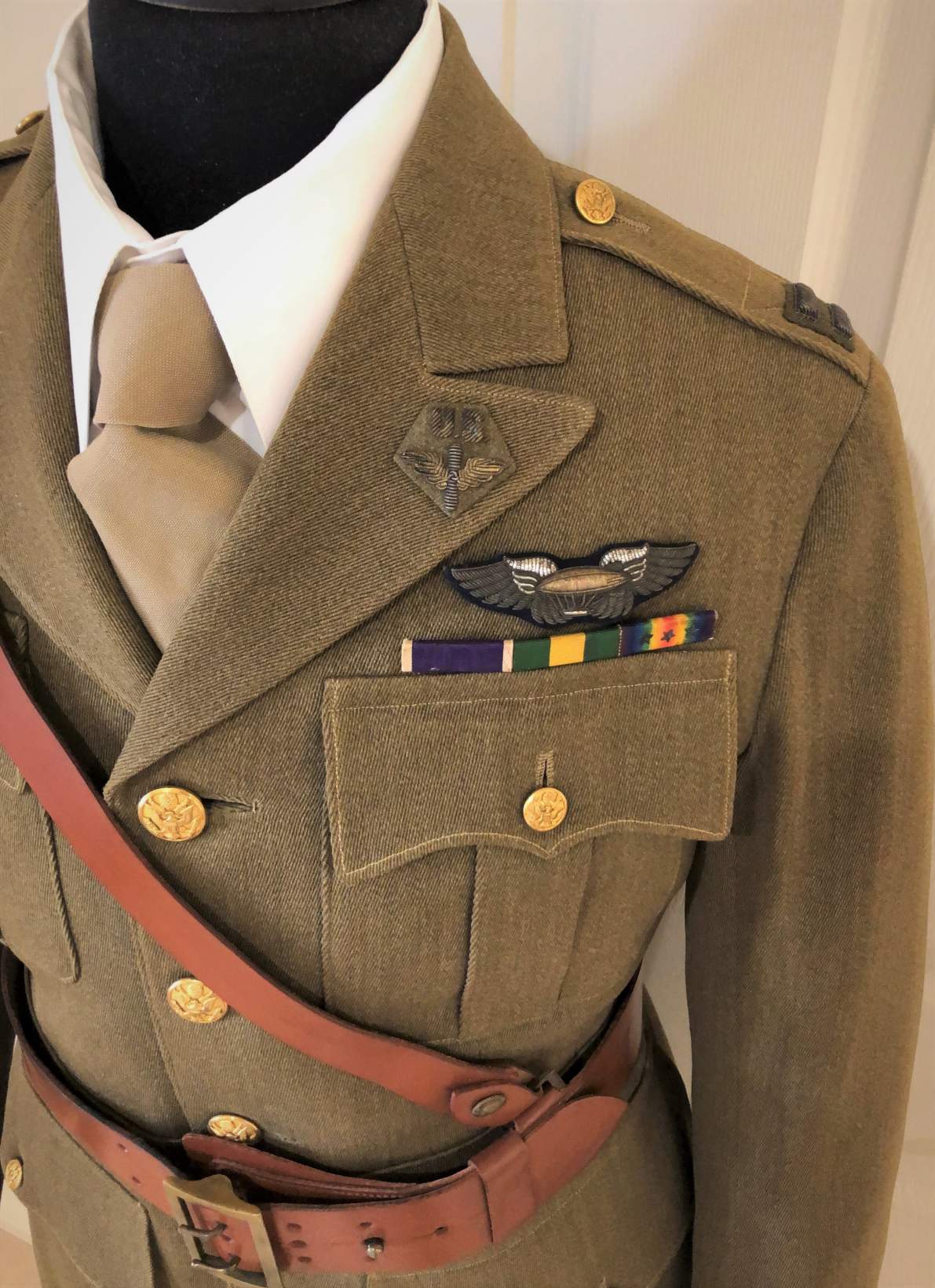The photograph captures a close-up, slightly top-right angled view of a black mannequin adorned with a vintage military uniform. The uniform features a thick, army-green overcoat adorned with brass buttons that run down the middle and secure a prominently cut flat pocket, reminiscent of western wear stylings. A white collared dress shirt and cream-colored tie lie beneath the overcoat. Nestled above the pocket, a distinct insignia of black wings with white detailing encircles a central emblem, likely denoting rank or affiliation. Additionally, a horizontal strip of colors, possibly representing a flag or the owner's colors, is positioned below the insignia. The ensemble includes dark bronzy shoulder epaulets, each marked with stripes. Completing the attire, a brown leather belt wraps around the waist, paired with a matching strap that crosses diagonally from the right shoulder, evocative of a historical officer's gun belt. The backdrop appears off-white, suggesting the setting is possibly indoors near a door.